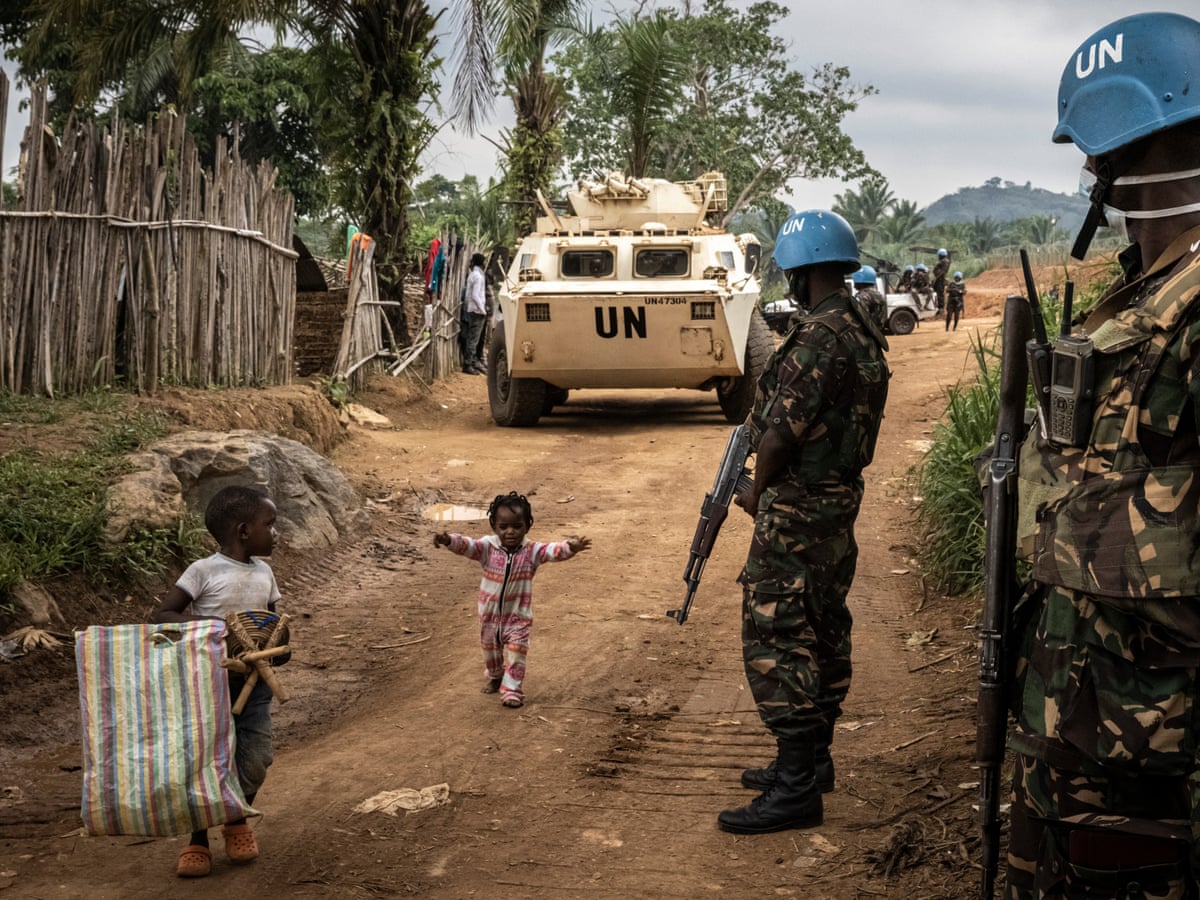In this outdoor scene, set on a dirt road amidst what appears to be an African or potentially Haitian landscape, two small Black children are captured at the center of the image. The little boy, dressed in a white t-shirt, dark pants, and peach-colored Crocs, carries a cloth-striped bag and possibly a wooden object. Beside him, a little girl wearing a pink, white, and orange onesie runs towards the camera with outstretched arms, as if seeking a hug.

Surrounding the children, there are numerous U.N. soldiers dressed in jungle camouflage fatigues. The soldiers, carrying AK-47 rifles and equipped with two-way radios, stand along the right side of the road and beside a troop transport vehicle marked "UN" in black letters. The vehicle, white in color and with features indicative of an armored transport or SUV, is parked further back on the road.

Additional details include a rustic wooden fence on the left side and a pickup truck with more soldiers in the background. Blue helmets with "UN" written in white letters are worn by the soldiers, who are seen climbing in and out of the vehicles. The backdrop of the image features hills, trees, and a cloudy sky, indicating a rural and possibly conflict-affected area.